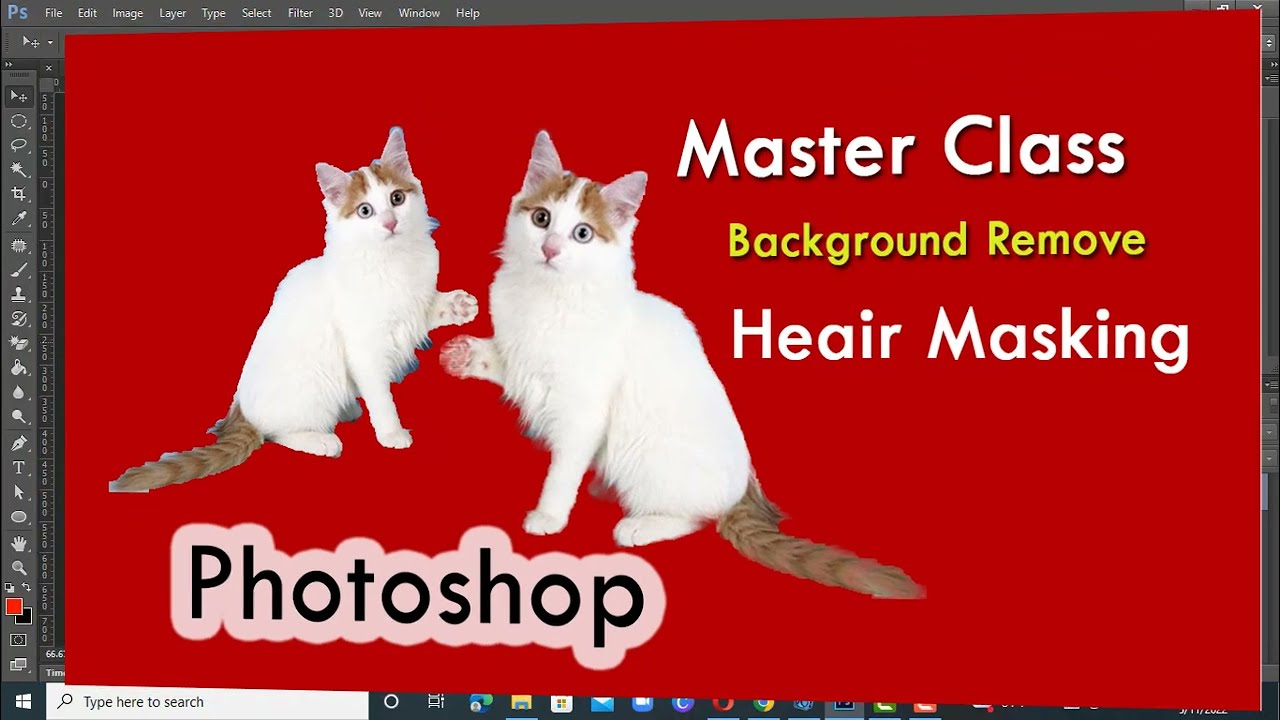In the image, we see a computer screen displaying Adobe Photoshop with a visible toolbar across the top that includes options such as File, Edit, Image, Layer, Type, Select, Filter, 3D, View, Window, and Help. The main focus is a graphic design piece, seemingly a flyer for a Photoshop tutorial, with a bright red background. The flyer prominently features two identical white cats with pointy ears facing each other; the cats are mirrored images with big, wide green eyes, brown markings near the top of their heads, and brown-striped tails with some white. Both cats have one paw raised. 

Adjacent to the cats, on the right-hand side, there is text, partly in yellow and partly in white, which reads "Masterclass Background Remove Hair Masking" (with "hair" misspelled as "heair"). Below the cats, the word "Photoshop" appears in black text, surrounded by a white outline that follows the shape of the text. The overall design is enclosed within the Photoshop window interface, emphasizing the tutorial's context within the software.